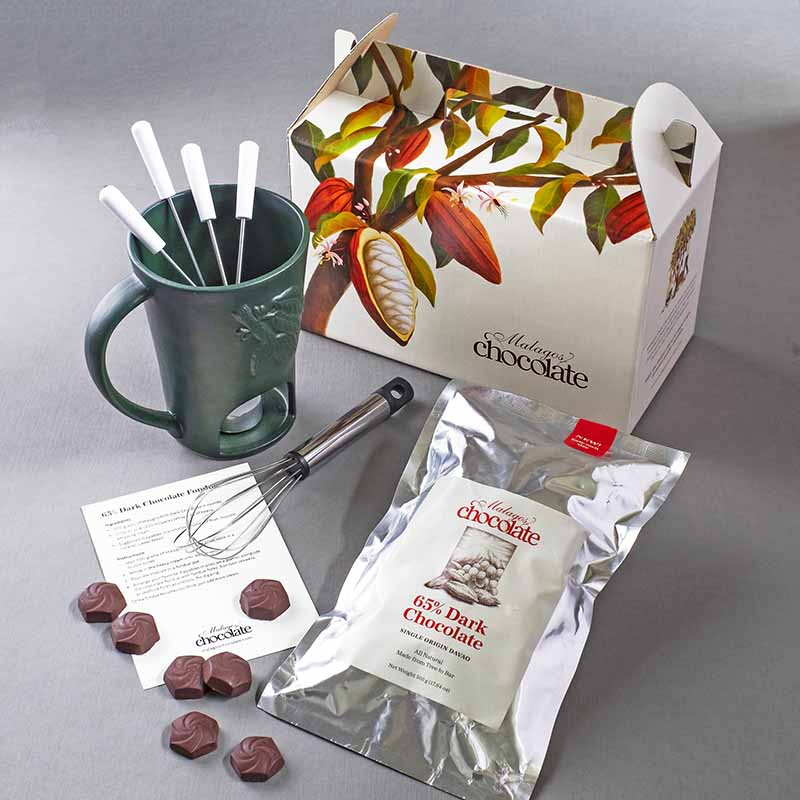This professional promotional photograph showcases a selection of Malagos chocolate products against a clean, gray background. Dominating the rear left section of the image is a green cup filled with white-handled stirrers and a mini whisk lying in front. To the upper right, a beige cardboard box adorned with an illustration of a cocoa plant prominently displays "Malagos chocolate" in cursive. Adjacent to this, in the lower right, sits a silver bag labeled "Malagos chocolate" with a red sticker indicating 65% dark chocolate. Scattered below on the left are about seven pieces of hexagon-shaped dark chocolate, arranged nearby a recipe card, tying the photographed items together as a cohesive set of chocolate-related products. Each element is meticulously placed to highlight the brand and its offerings for potential buyers.